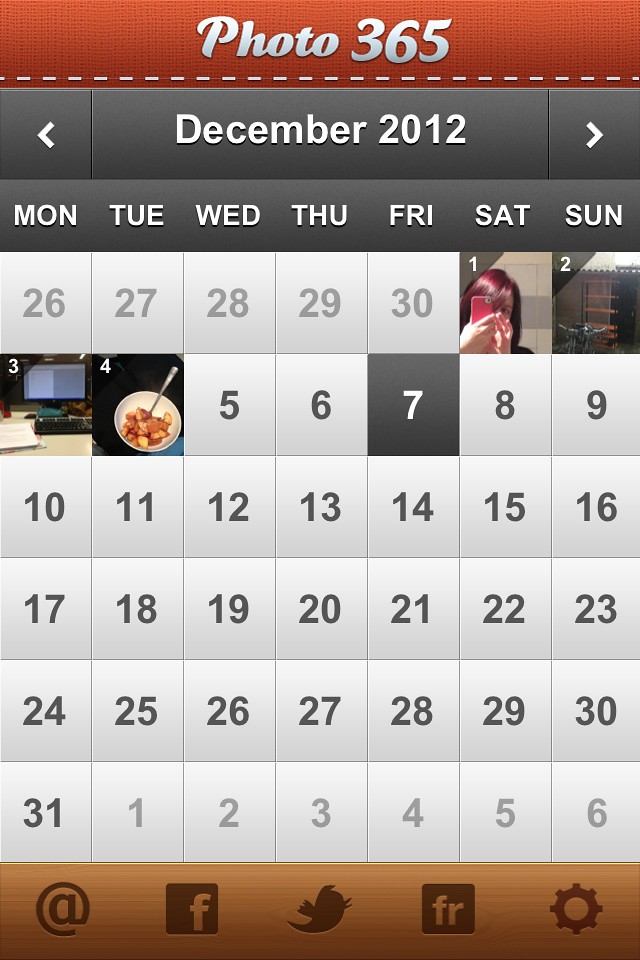The image depicts a calendar with the month of December 2012 clearly shown. At the top of the calendar, the text "Photo 365" is prominently displayed. The calendar follows a Monday-through-Sunday format, from left to right. At the bottom of the calendar is a stripe that contains the text "at" along with several emblems: the Facebook logo, Twitter logo, the "FR" symbol, and a gear icon indicating settings or options.

The calendar dates span from November 26th to January 6th. On December 1st, the date block features a picture of a woman peeking around the corner of her cell phone. December 2nd shows another image, which is not as easily identifiable but appears to be a performer with arms outstretched in front of a microphone. On December 3rd, the image within the date block seems to depict a media room or media center. December 4th showcases a bowl of fruit, including strawberries. The date block for December 7th is blackened with no image present. The remaining dates are displayed on a neutral background with no additional imagery.